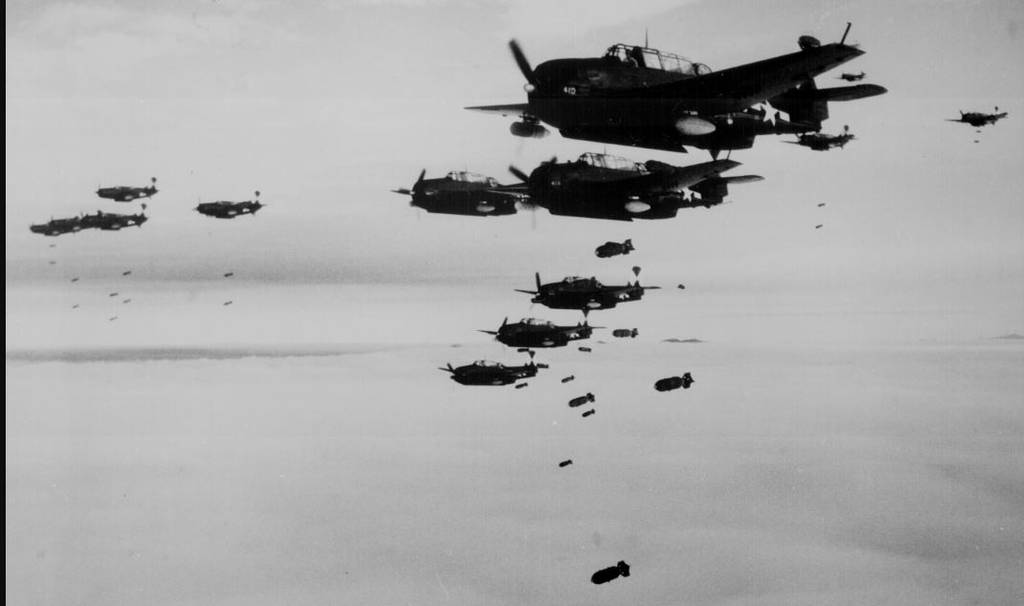This black and white, grainy photograph likely dates back to World War II, portraying a dramatic aerial scene. A total of 12 old fighter planes, identifiable by their propellers and the stars with lines on each plane's side, soar through a cloudy sky in a tight formation. All planes seem to be traveling to the left, with several of them visibly dropping bombs below. The photograph's vintage quality, combined with the gloomy, overcast sky and absence of any text, amplifies the historical and somber essence of the image.